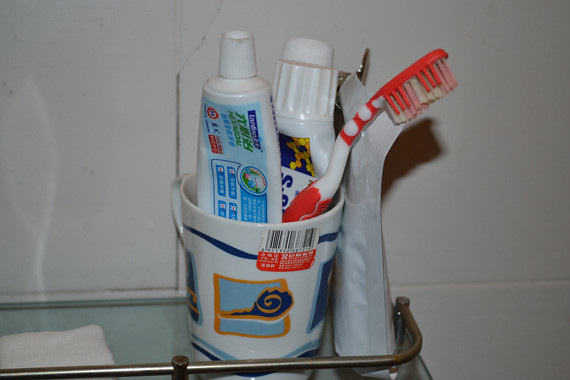The close-up image captures a bathroom scene with a focus on a small glass shelf that features an aluminium metal trim, approximately a centimeter or so tall, finished in a bronzish color. The backdrop is a tiled wall with white ceramic tiles, with just three or four tiles visible due to the proximity of the shot. 

Sitting on the glass shelf is a white ceramic mug adorned with blue, light blue, yellow, and orange patterns. Notably, the mug still has its store UPC barcode sticker attached, with a red section indicating product information. Inside the mug are two tubes of toothpaste; one prominent tube is light blue and white, accompanied by a second tube with an unusually wide lid. Also within the mug is a red and white toothbrush that has an orange tip, a white centerpiece, and a pinkish-reddish handle. Positioned near the mug, on the very edge of the shelf, there's a sachet-like item.